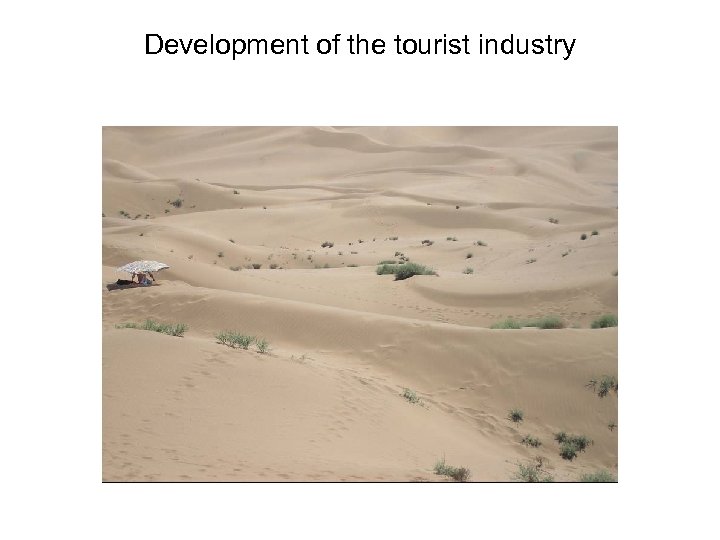This image captures a sprawling desert environment dominated by undulating sand dunes, with little vegetation sparsely distributed across the landscape. The sand appears to be hilly and textured with layers, creating various contours and mounds. Small patches of spiky green grass peek out intermittently from the sand, adding slight bursts of color to the tan and brown expanse. There are also footprints and markings in the sand, hinting at the presence of life amidst this otherwise barren setting. On the left side of the image, a vacationer or tourist is seated on a towel under a light gray umbrella, which provides them shade from the sun. This scene ties into the text at the top of the image, which reads "Development of the Tourist Industry," suggesting a focus on encouraging tourism in desert areas. The photo features a color palette of blacks, whites, tans, browns, greens, and blues, contributing to its stark yet picturesque depiction of desert solitude.